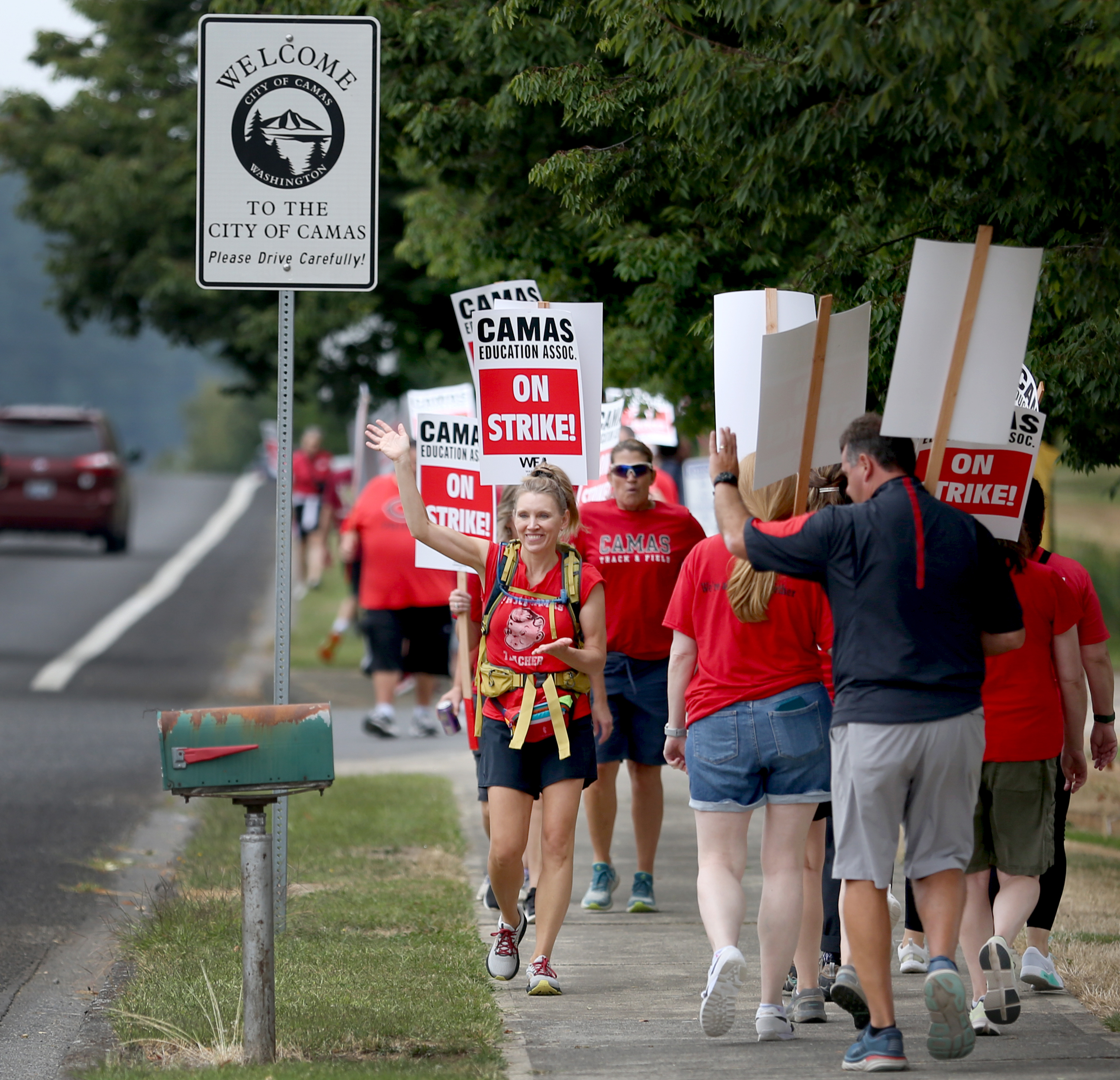In this photograph, we see a semi-rural, suburban scene featuring an active picket line on the sidewalk to the right of a road. The road, located on the left side of the image, has a white boundary line and a red car traveling midway down its length, which appears somewhat blurry. The sidewalk is more in focus, particularly in the center but not in the background. On the right side of the image, people are wearing red crewneck t-shirts and shorts, indicative of a warm day, and walking up and down the sidewalk with picket signs reading "Kamas Education Association on strike."

In the foreground, between the street and the sidewalk, there is a green mailbox with some rust on its top, mounted on a gray pole. Behind the mailbox, a prominent sign reads, "Welcome to the City of Kamas, C-A-M-A-S. Please drive carefully," with an icon of mountains and trees and "Washington" underneath. The top portion of the picture features trees spanning from the top left to the right. The protesters, part of the Kamas Education Association, are waving to passing traffic, engaging with their surroundings as they walk along the sidewalk.